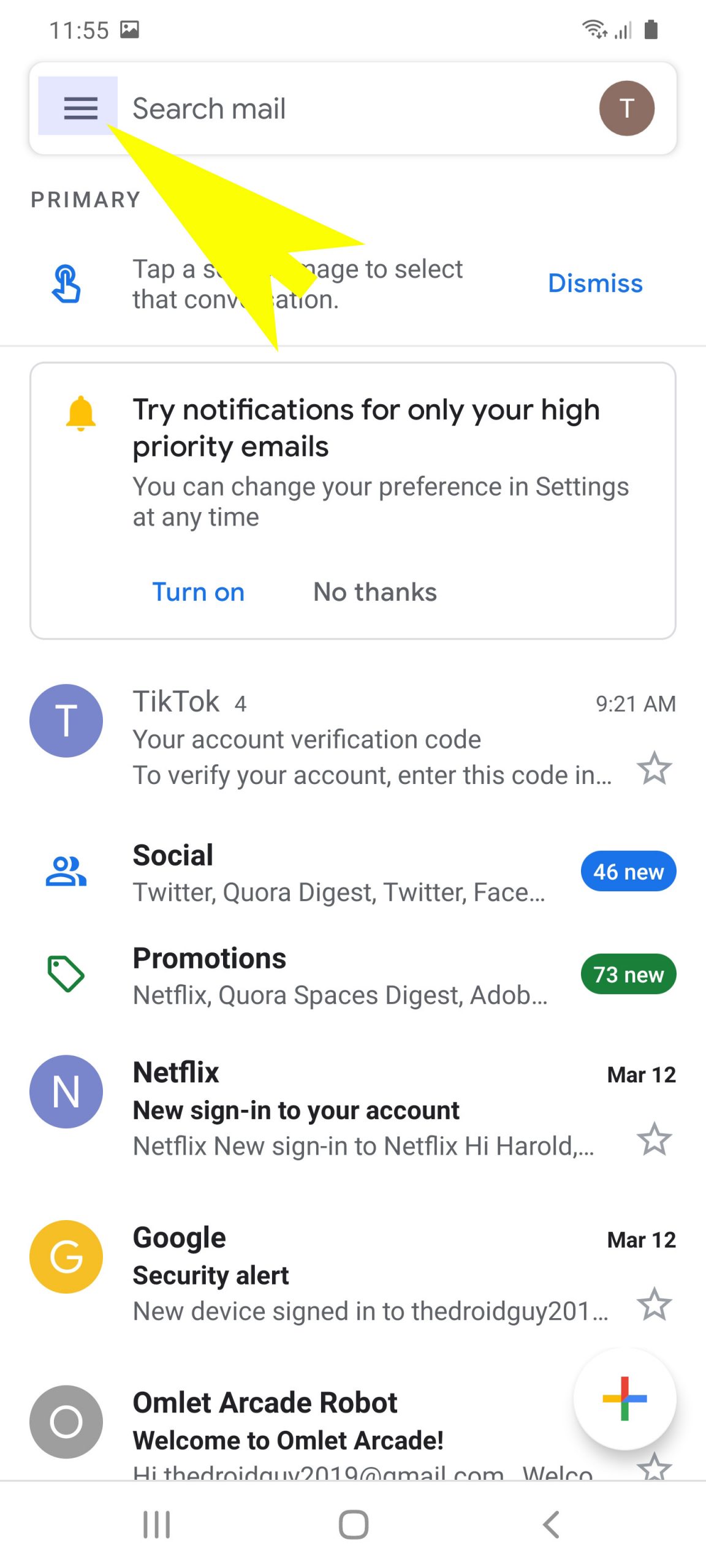The image is a screenshot from a phone displaying someone's email inbox. The top of the screen shows the time as 11:55, with icons indicating a connected WiFi and a full battery. A large yellow arrow is pointing at three horizontal lines in the search mail tab, suggesting a navigation menu. Next to this, the letter "T" is visible, indicating a link to the user's profile.

In the "Primary" tab, a notification bar encourages the user to "Try notifications for only your high priority emails," with options to "Turn on" in blue and "No thanks" in gray. The first email listed is from TikTok, received at 9:21 AM, indicating an account verification code. Right next to it is a small star icon.

Below the Primary tab, the "Social" tab features icons of two blue people and contains emails from platforms like Twitter, Quora Digest, and Facebook (truncated to "Face").

Further down is the "Promotions" tab, marked by a price tag icon. It contains emails from companies like Netflix, Quora Spaces Digest, and Adobe, with a notification of "73 new" emails. An email from Netflix, dated March 12th, addresses a user named Harold regarding a new device sign-in. 

The next email, from Google, features an orange "G" and alerts of a new device signing into an account associated with "the droid guy." Finally, an email from Omelette Arcade, marked with an "O," welcomes the user to the service.

At the bottom of the screenshot, there are icons representing standard email functions, such as lines, a square, and an arrow.